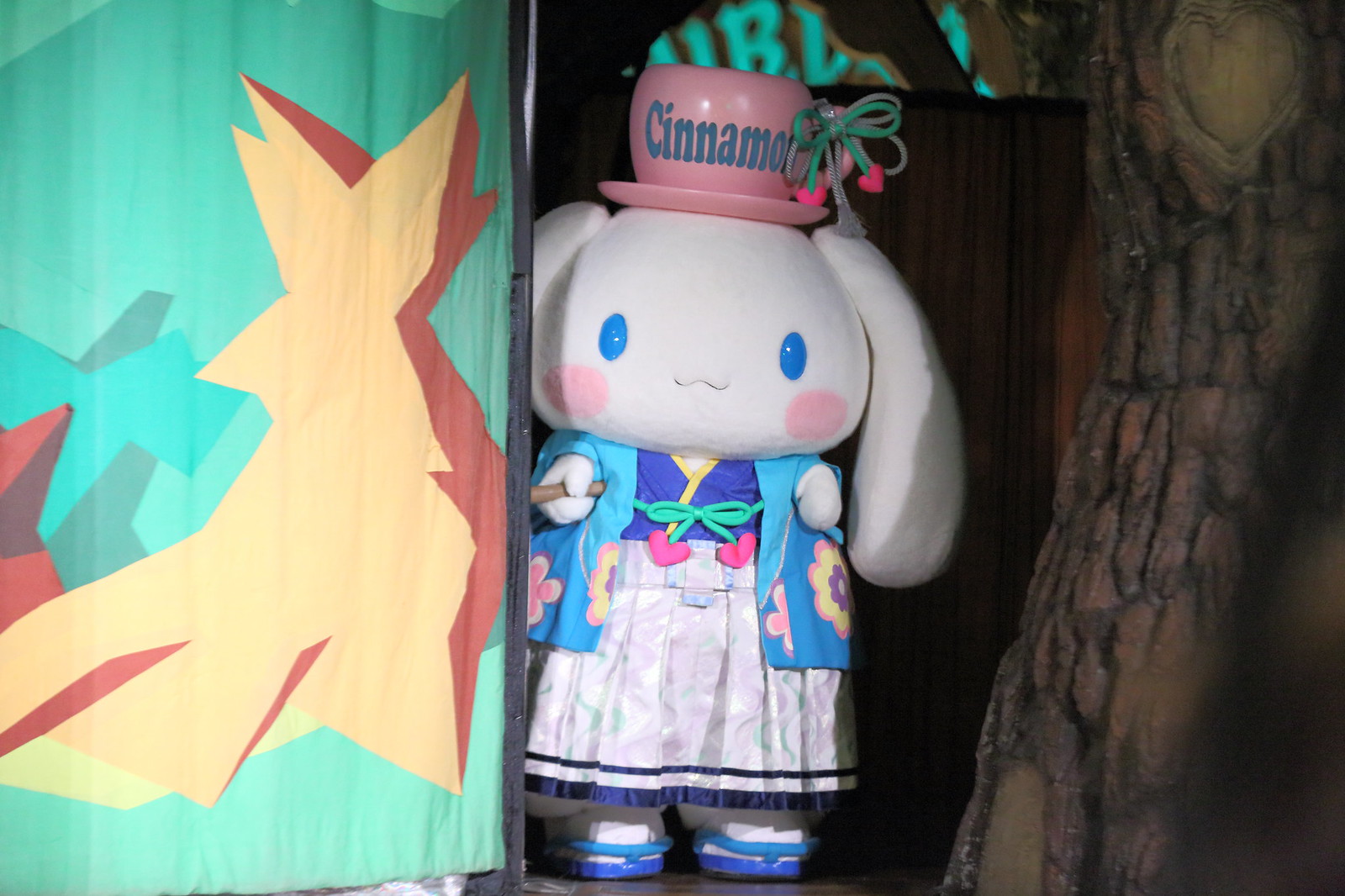In this vibrant and whimsical indoor scene, a central stuffed animal stands out - a rabbit with long, white ears and glossy blue eyes dotted with pink cheeks. This character, suggestive of a Japanese anime influence, is adorned with a plethora of detailed attire: a blue floral jacket over a purple and yellow shirt, with a green string tied in a bow with heart ends. It wears a soft pink dress accented with a blue border and dons matching blue shoes. Atop its head, it balances a pink teacup inscribed with the word "cinnamon."

To the left of the rabbit, there is a piece of fabric featuring an intricate design, while on the right, a wooden structure or possibly a tree trunk with a carved heart can be seen. Adding to the whimsical setting, a green sign with yellow and orange graphics is also present. The image is filled with a palette of light blue, red, yellow, green, pink, blue, and purple hues, further enhancing the lively atmosphere. The background suggests a scene akin to a puppet show or a playful indoor display, bringing a delightful and animated feel to the image.